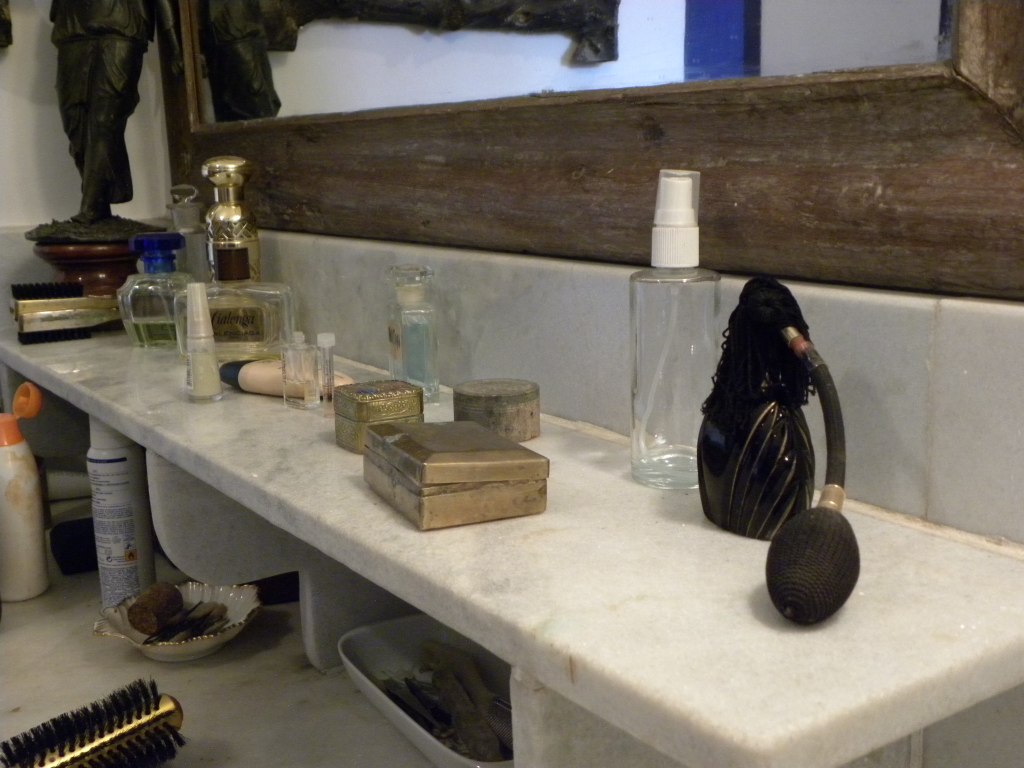The image showcases a close-up of an elegant shelf crafted from white stone, accentuated by delicate gray veins. Positioned in the far upper left corner of the shelf is a statue. Following the statue, a collection of perfume bottles is neatly arranged, interspersed with a couple of travel-sized toiletry bottles reminiscent of those found in hotels. Adjacent to them are three small jewelry cases. On the right, an empty spray bottle with a white cap is placed, bookended by a black perfume bottle with its spray mechanism located at the very bottom.

Beneath the main shelf, on the left side, a white bottle with an orange lid is visible, with another white bottle situated to its right. Directly below these bottles, a small white dish contains several assorted items, while a portion of a round gold hairbrush peeks into the frame from the lower left corner. An additional dish, resting directly under the shelf, holds a mysterious unidentifiable object. Crowning the top of the frame, the bottom part of a wooden-framed mirror can be seen, adding a final touch of sophistication to the scene.